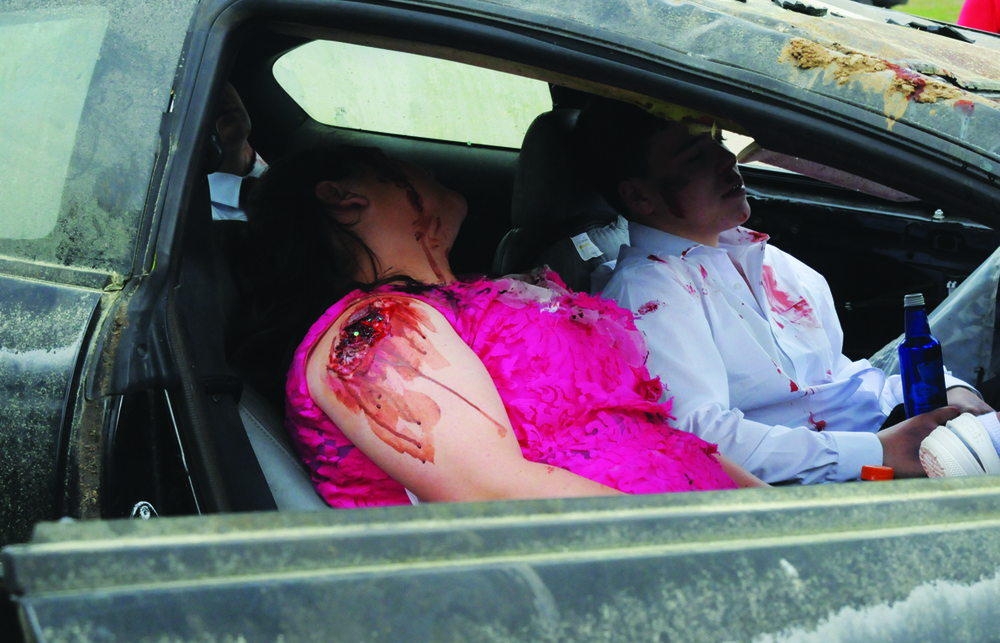This photograph captures a harrowing scene inside a car with its door open. There are three individuals visible: a woman in the passenger seat, a man in the driver's seat, and a man in the backseat. All three appear to be Caucasian with brown hair and dressed in formal attire. The woman in the passenger seat is wearing a pink, maroon-colored dress and has visible wounds, with blood trickling down her cheek and neck. The man in the driver's seat, dressed in a white shirt and grayish pants, is holding a blue bottle with a white tip in his right hand. His shirt is stained with what appears to be blood, though no visible wounds are noted. The man in the backseat is wearing a suit and tie. The car's exterior is black and covered in brown dirt, adding to the eerie and grim atmosphere. Although the scene looks quite realistic, the blood and wounds could suggest that this was staged, perhaps for a Halloween event.